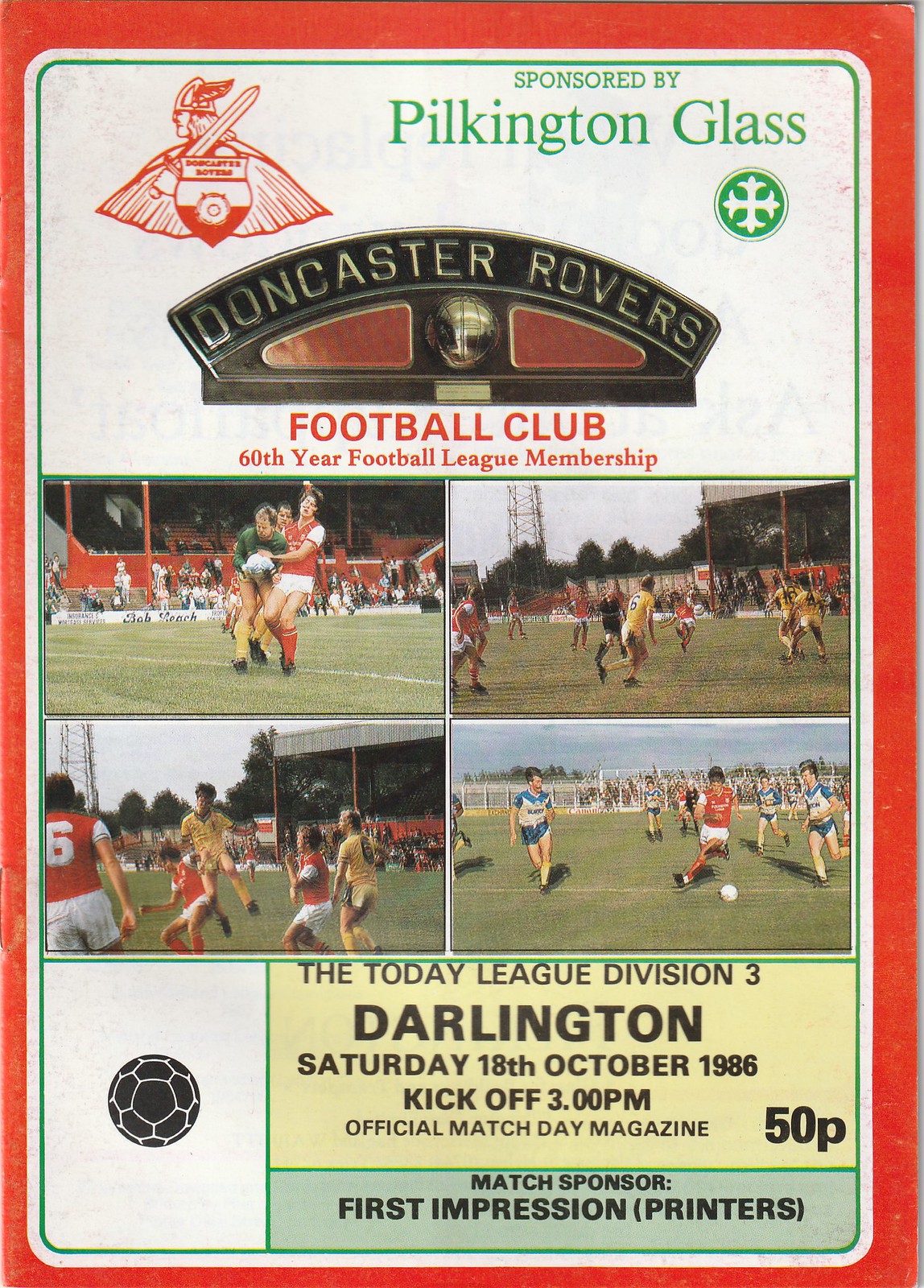The image is an advertisement for a soccer match featuring a vibrant red background. At the top, there is an icon resembling a Viking with a shield, sword, and winged helmet, looking off to the side. To the right of this icon, green text announces the sponsorship by Pilkington Glass. Directly below, in red text, it celebrates Doncaster Rovers Football Club's 60th year of Football League membership. The center of the ad features four action-packed photos of football players, mainly in red and white jerseys, indicative of the Doncaster Rovers, competing against teams in various other colored jerseys like blue, yellow, and green. Below these images, finer details are provided: a logo of a soccer ball is positioned on the bottom left, adjacent to text detailing the event—Today League Division III versus Darlington, scheduled for Saturday, 18th October 1986, with a kickoff at 3 p.m. The magazine is labeled as the official match day publication, priced at 50 pence, and mentions the match sponsor, First Impression Printers. The entire layout is framed with a white and green border, further enhancing its vibrant presentation.